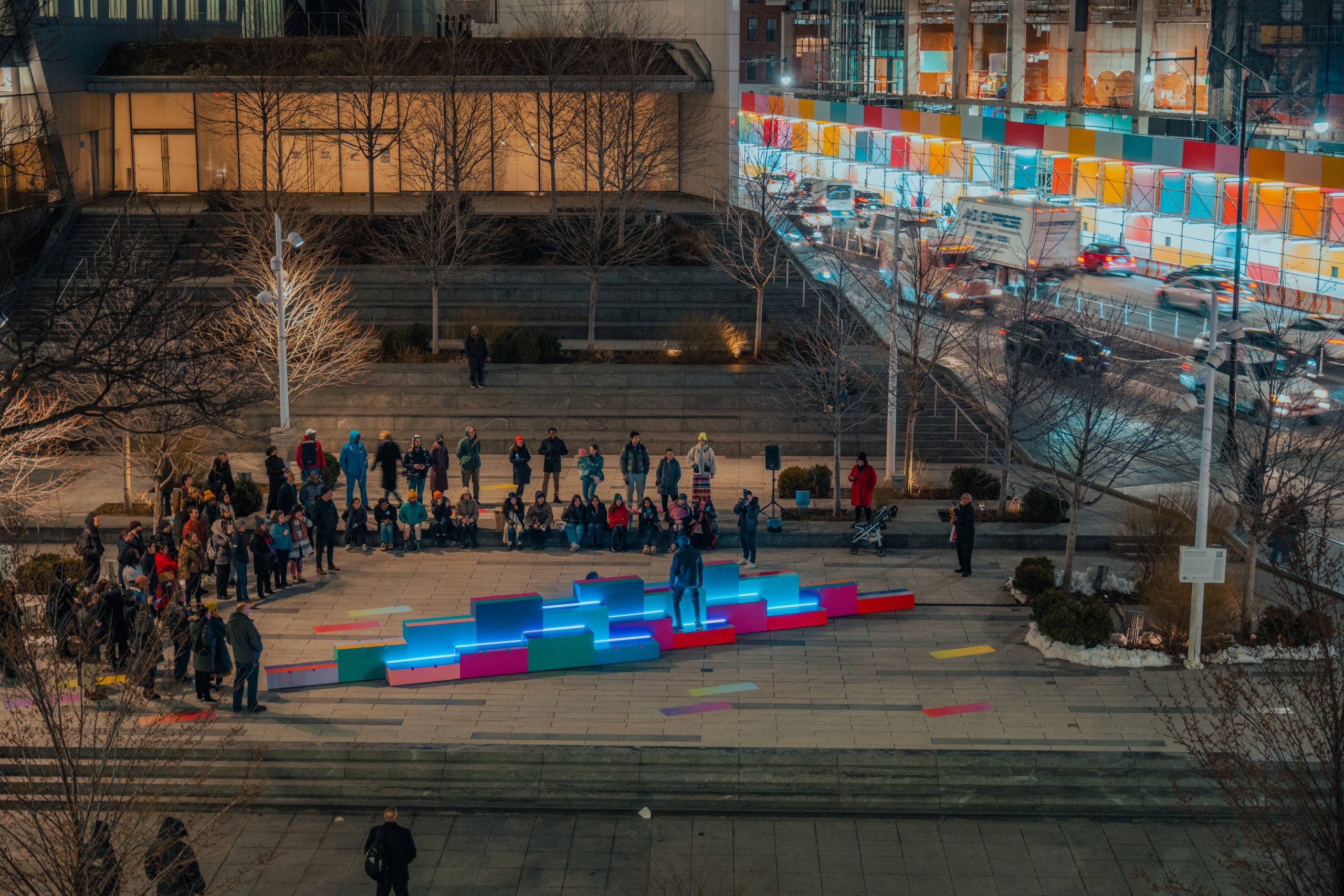The image depicts a bustling urban scene at night, featuring a vibrant public art display or street performance. Central to the image is a raised platform composed of multicolored rectangular steps, illuminated by fluorescent blue lights. These steps range in colors including pink, raspberry, green, aqua, teal, and red. A man dressed in dark clothing stands atop a red step, surrounded by an attentive crowd forming a semicircle around the platform. The crowd is gathered on stone pavement, encircled by shrubs and trees, with a light dusting of snow on the ground.

In the background, two buildings are visible. The one directly behind the crowd is large and gray, while the one to the right is decorative and colorful, adorned with siding in shades of pink, green, blue, red, orange, and white. This structure appears to have scaffolding on it. Off to the right of the image, a busy city street with passing cars can be seen, adding to the lively nighttime atmosphere. Street lamps and lights from the surrounding buildings illuminate the scene, capturing the essence of this urban evening gathering.